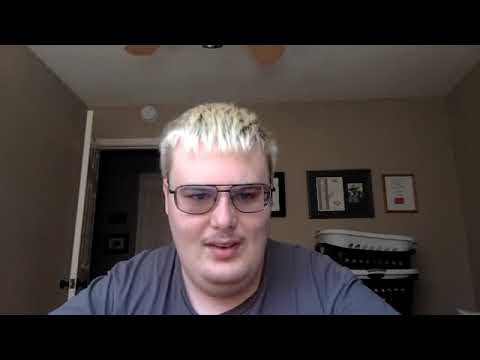The image depicts a slightly chubby young white man with platinum blonde hair, cropped short. He sports thin black-framed eyeglasses and has a bit of stubble on his mustache, and his moustache has hints of his natural brown hair color. He wears a bluish-gray t-shirt and appears to be seated, possibly at a desk, looking directly into a webcam, suggesting that he might be on a Zoom call or recording a video for streaming purposes. Behind him, a room is visible with greenish-beige walls adorned with three picture frames. To the right of the frames, there's a stack of plastic laundry baskets in varying colors – white, black, and blue. An open door can be seen on the left side of the room, with the tips of ceiling fan blades peeking into the frame above his head.